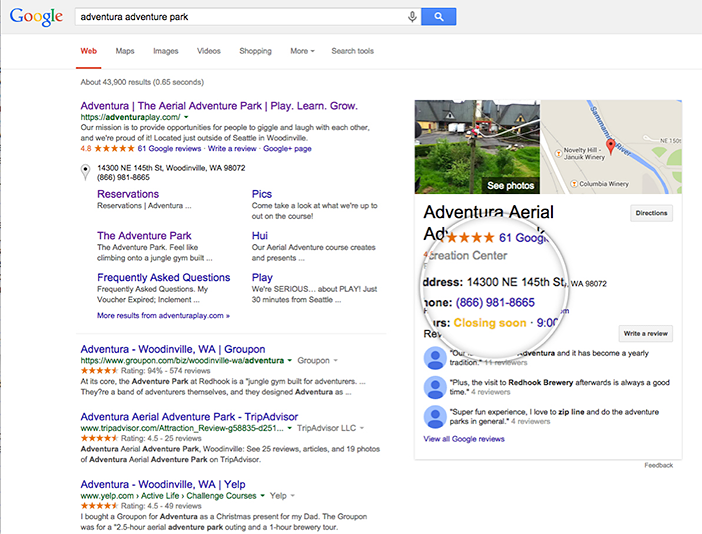Screenshot of a Google search for "Adventure Adventure Adventure Adventure Park". The search bar displays the repeated phrase, flanked by the voice search icon and search button. The menu options "web", "maps", "images", "video", "shopping", and "more search tools" are visible with "web" selected. The search yielded approximately 43,900 results in 0.65 seconds. The top link directs to "Adventura, the Aerial Adventure Park - Play, Learn, Grow" at AdventuraPlay.com. Below it are links to the reservations page and the Adventure Park page, both previously visited. Subsequent results include references to Adventura, Woodinville, Washington, listed on TripAdvisor and Yelp. On the right side, information about "Adventura, Aerial Adventure Park" is highlighted, seemingly zoomed in by a built-in Windows magnifier or editing tool. The zoom focuses on the phone number (866-981-8665), partial address (14300 NE 145th Street, Washington), and indicates the park is closing soon, likely at 9 p.m. The city name is truncated.